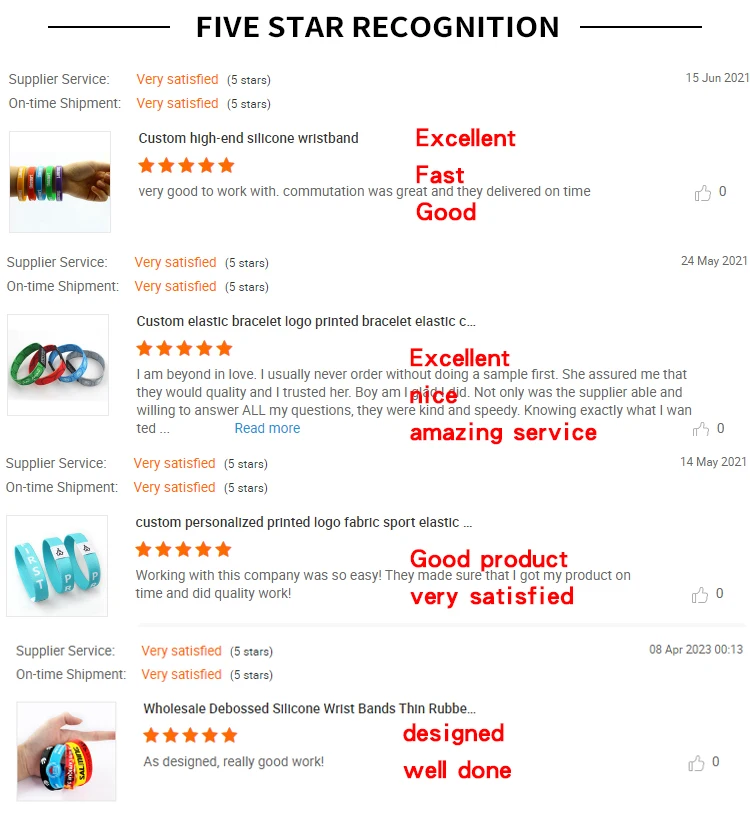The image features a clean white background with a prominent heading at the top in black capital letters that reads "5 STAR RECOGNITION." This title is flanked by horizontal bars on either side. Below the title, four different products are displayed in a vertical list format, each accompanied by a detailed description, star rating, and user review. 

Each product is illustrated with an image to the left and a comprehensive description to the right. The first product is labeled as "Custom High-End Silicone Wristband," boasting a 5-star rating. The user review for this item reads, "Very good to work with. Communication was great and they delivered on time." Complementing the review are red text superlatives that emphasize "Excellent," "Fast," and "Good."

The second product is identified as "Custom Elastic Bracelet Logo," described further as a printed elastic bracelet. Like its predecessor, it comes with a star rating and a detailed text review. 

The third product on the list is the "Custom Personalized Printed Logo Fabric Sport Elastic," also featuring a star rating and user feedback.

The final product is "Wholesale Debossed Silicone Wristbands, Thin Rubber," similarly accompanied by a star rating and a review.

Each product entry is accentuated with red-lettered positive attributes such as "Excellent," "Nice," "Good Product," and "Very Satisfied," providing a quick, visual endorsement of their quality and customer satisfaction.